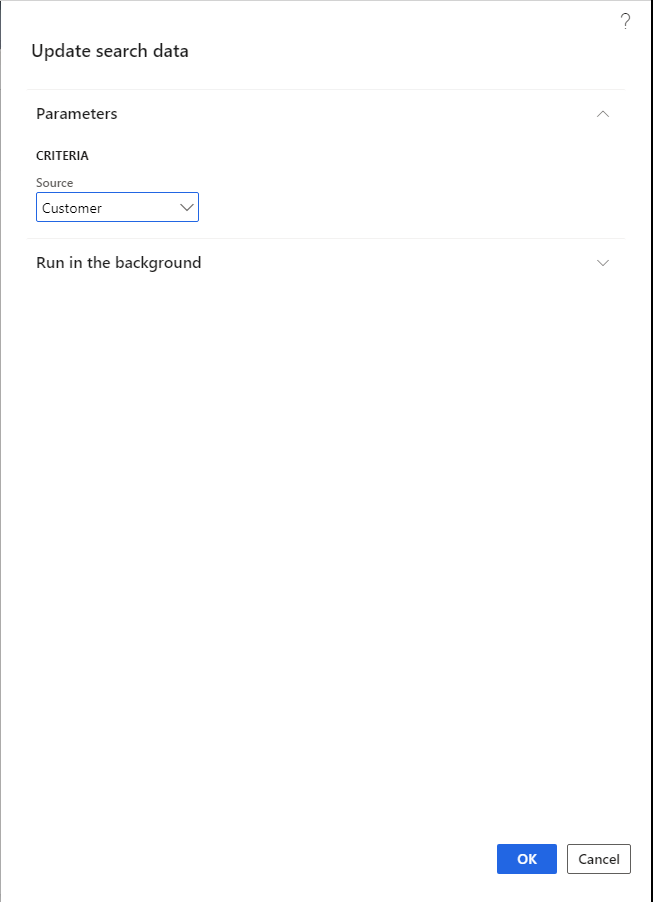The image captured from a device screen showcases a rectangular interface featuring several sections. In the top left corner, the text "Update Search Data" is prominently displayed. Below a faint gray line, a section titled "PARAMETERS" is seen, with the heading "CRITERIA" marked in bold black capital letters. Directly underneath, the word "Source" appears in smaller print, with only the 'S' capitalized. 

Further down, a blue rectangular drop-down menu labeled "Customer" is visible, indicating selectable options. Another faint gray separator line follows, under which the phrase "Run in Background" is displayed. On the far right of the same section, a downward pointing arrow contrasts with the previously mentioned upward pointing arrow in the "Parameters" section.

In the upper right corner of the interface, a gray question mark icon is positioned. At the very bottom of the screen, there are two buttons: a blue "OK" button and a white "Cancel" button.